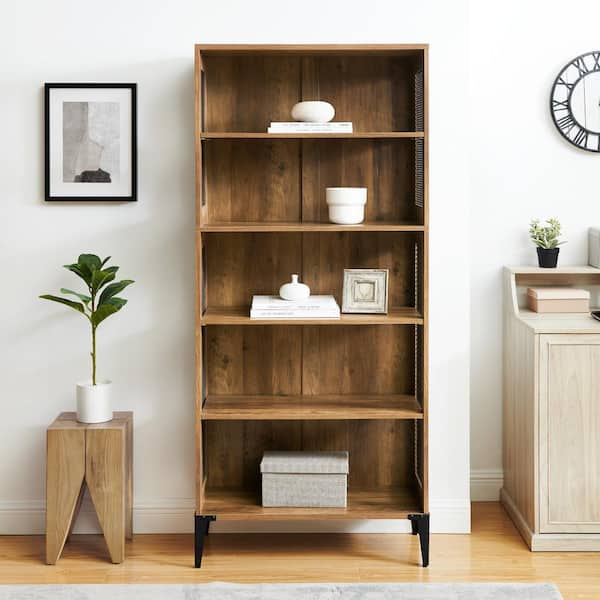This image is a photograph of a contemporary, indoor room, featuring minimalist design elements and modern furniture. The central piece in the room is a wooden, five-shelf bookcase with stained brown wood and four black metal legs. Each shelf displays specific decorative items: the bottom shelf holds a decorative box, the third shelf up has two white books, a white vase, and a white picture frame, the next shelf houses a white ceramic pot, and the top shelf features two stacked white books and an oval white ceramic object. 

To the left of the bookcase is a small, modern side table made of light brown wood with uniquely designed legs that are wider at the top and narrower at the base. On this table sits a white planter containing a slender-stemmed plant with broad green leaves. Hanging above the table is a simple black-and-white photograph in a minimalist style. 

To the right of the bookcase, partially visible in the photograph, is a piece of stained white wooden furniture, possibly a desk, holding a small plant in a black pot and some papers or a shadow box. Completing the scene, there is a glimpse of a black-and-white clock with Roman numerals positioned above the desk. The entire setup is arranged against a pristine white wall, and the floor is of medium-toned wood, all contributing to the room's contemporary aesthetic suitable for a catalog or website display.